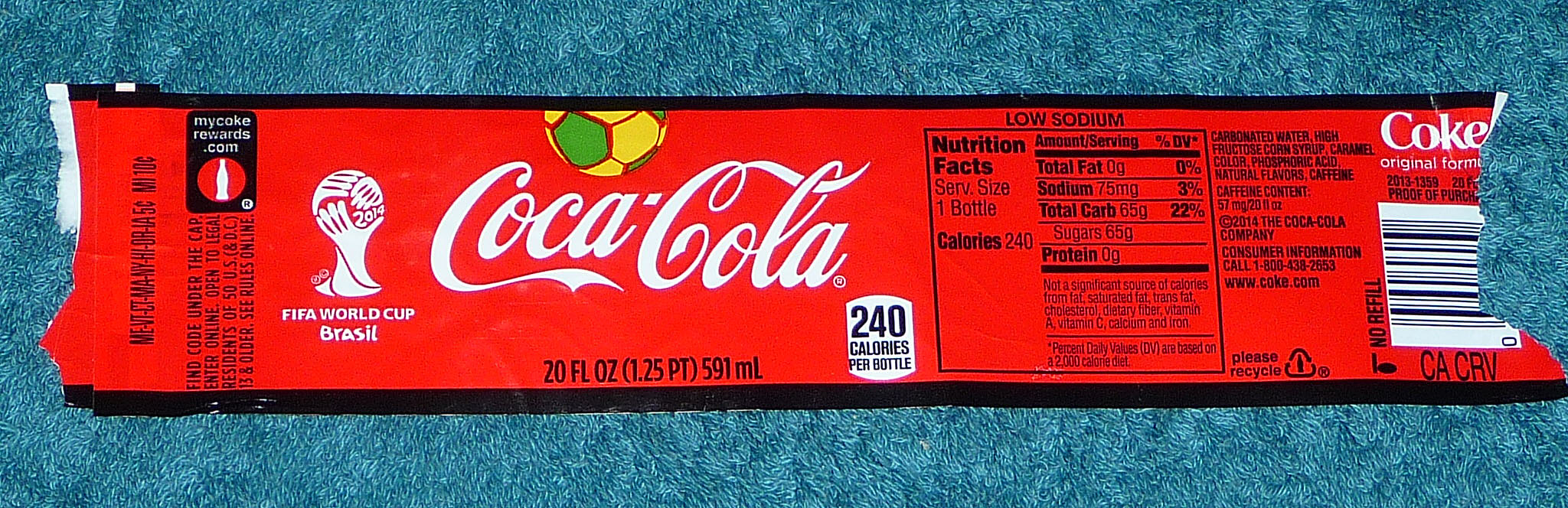The image showcases a Coca-Cola label that appears to have been peeled off from a bottle. The label prominently features the branding for the FIFA World Cup Brazil, with "Coca-Cola" written in white letters. The label specifies that the bottle contains 20 fluid ounces (591 milliliters) and indicates 240 calories per bottle. A colorful soccer ball, primarily yellow and green, adds to the World Cup theme. Additionally, there is a section with nutritional information, part of a barcode, and the World Cup logo in white, displaying the year 2014.

The label also includes text about "My Coke Rewards" and instructions on recycling the bottle for a small monetary value. The background of the label is mainly red, accented with black stripes. At the bottom, there is a reminder to "Please Recycle," along with a detailed list of ingredients. The overall design emphasizes the festive and international spirit of the 2014 World Cup held in Brazil.